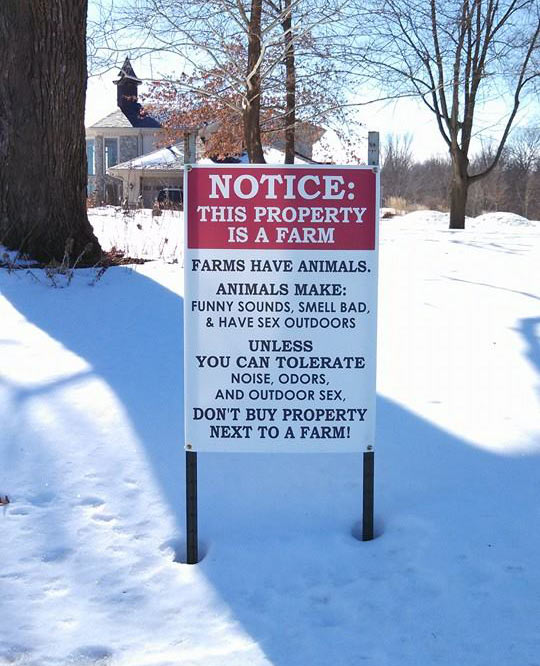In the foreground of this sunny, snowy outdoor scene, a prominent rectangular sign made of canvas commands attention. The sign features a red banner at the top with bold white letters declaring, "Notice: This property is a farm." Below, in black text, it humorously warns: "Farms have animals. Animals make funny sounds, smell bad, and have sex outdoors. Unless you can tolerate noise, odors, and outdoor sex, don't buy property next to a farm!" The landscape is dotted with several trees, including a significant large tree trunk situated in the upper left. In the far distance, slightly off to the left, there is a sizable white house with a stone facade, large windows, and a dark-colored roof, along with an attached garage. The clear, sunny sky illuminates the rustic setting, highlighting the blanket of snow that covers the ground and accentuates the peaceful yet candid nature of this countryside property.